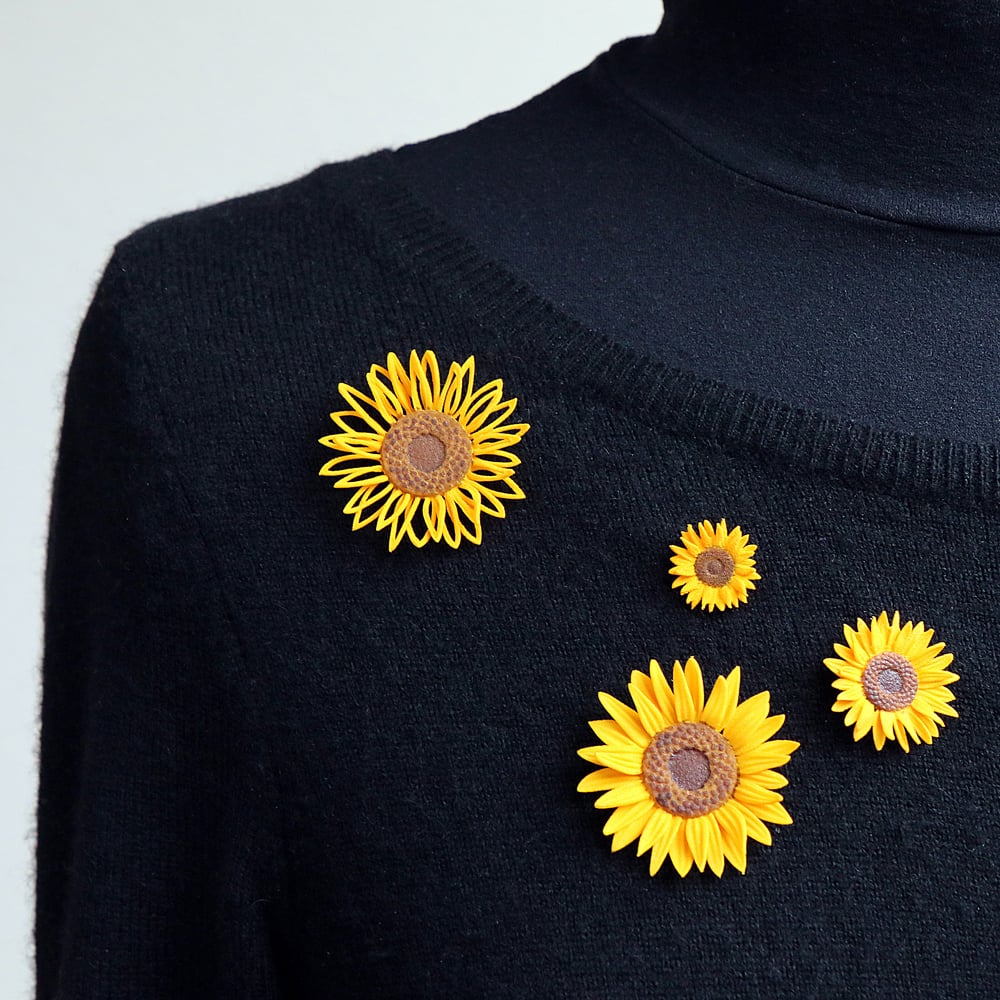The image features a vintage black sweater displayed on a mannequin, showcasing intricate detailing typical of fashion from 50 to 60 years ago. The sweater features a scooped, ribbed neckline which reveals a dark blue turtleneck worn underneath. Adorning the front shoulder area of the sweater are four medium-sized, vibrant yellow sunflowers, likely crafted from soft cloth or plastic. These flowers, characterized by their prominent brown centers, add a striking contrast to the dark fabric. The long sleeves and overall design suggest it could be an exhibit in a museum. The dominant colors in the image are black and yellow, with a hint of dark blue from the turtleneck underneath.